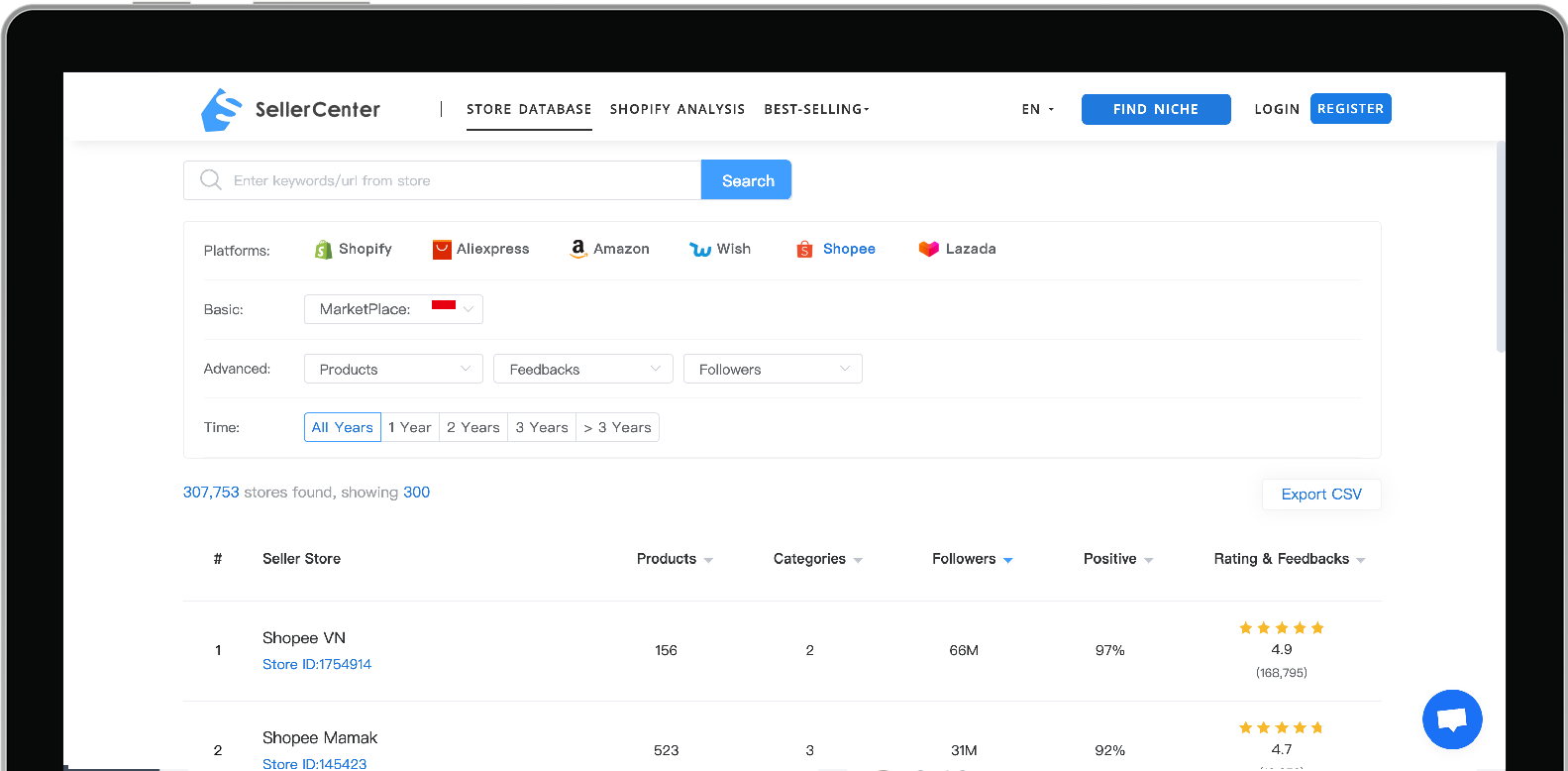In this screenshot, we are viewing a portion of what appears to be the top of a tablet or laptop screen, displayed in a horizontal orientation with its exterior framed in black. 

At the top of this visible section of the screen, there are two physical buttons on the device. Focusing on the screen display within this frame:

- **Upper right corner**: There is a prominent blue button labeled "Register" in white text.
- **To the left of this button**: Against a white background, the word "Login" appears.
- **Further left**: Another blue action button is visible with the text "Find Niche."

**Upper left corner**: Features a logo shaped like a light blue pencil with a white 'S' inscribed over it. Next to the logo, the words "Seller Center" are displayed.

**Top banner of the website**: Displays various options from right to left:
- "Store Database" in black text, underlined.
- "Shopify Analysis"
- "Best Selling"

Immediately beneath this banner is a white search bar accompanied by a blue action button labeled "Search."

This detailed caption captures the interface and elements visible on the screen, lending clarity to the viewer regarding the layout and functionality presented in the screenshot.